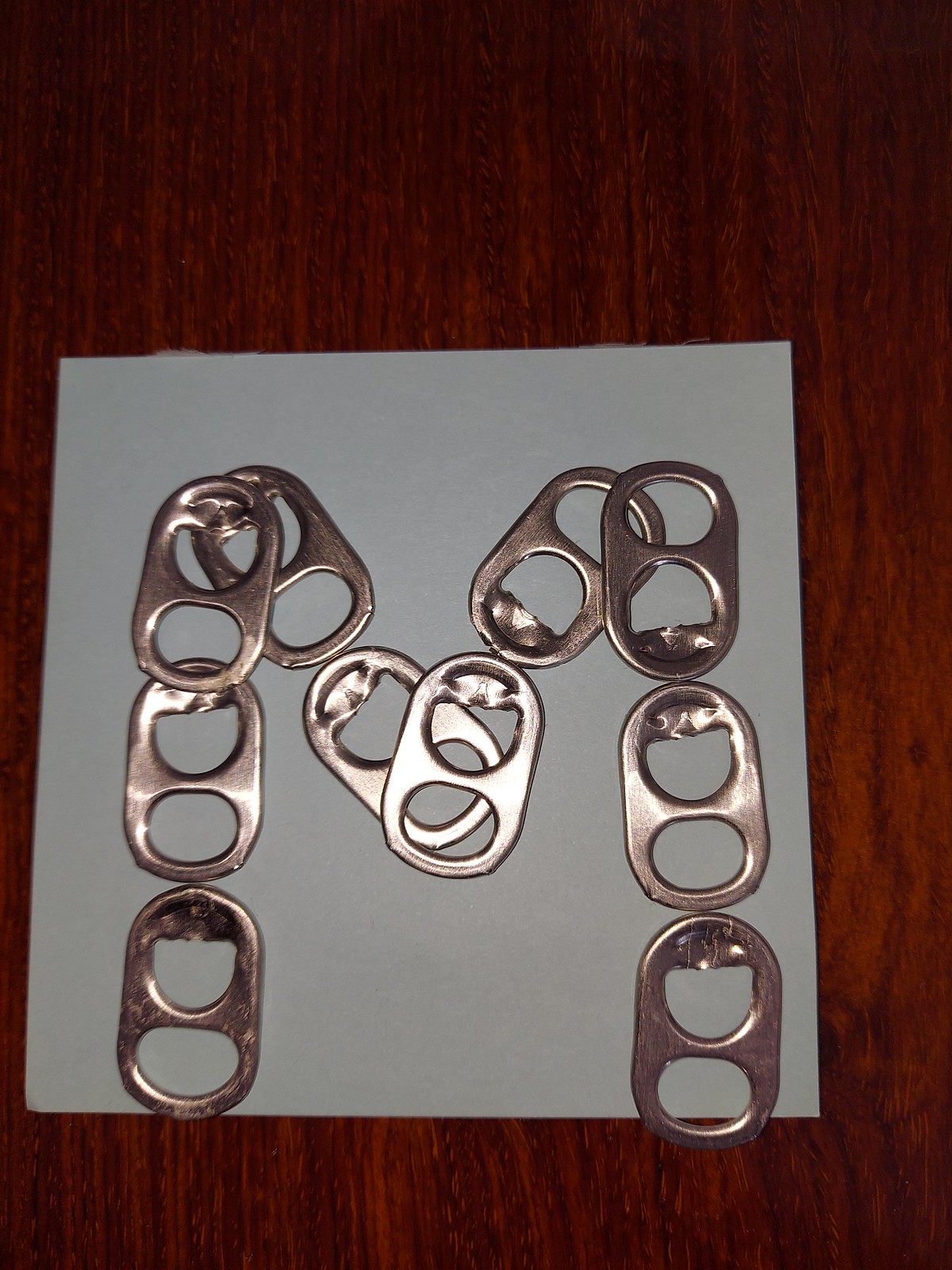This is a detailed photograph of shiny, oblong, aluminum can pull tabs, each featuring two holes, one above the other. There are approximately ten to thirteen of these old-fashioned soda can tabs arranged meticulously to form the shape of an uppercase letter 'M'. This arrangement is laid out on a blue or gray sticky note, which contrasts vividly against a dark brown wooden surface with visible grain. Some of the tabs overlap each other, enhancing the intricacy of the design. The metallic tabs, while largely polished, bear light scratches, adding a touch of texture to their appearance.